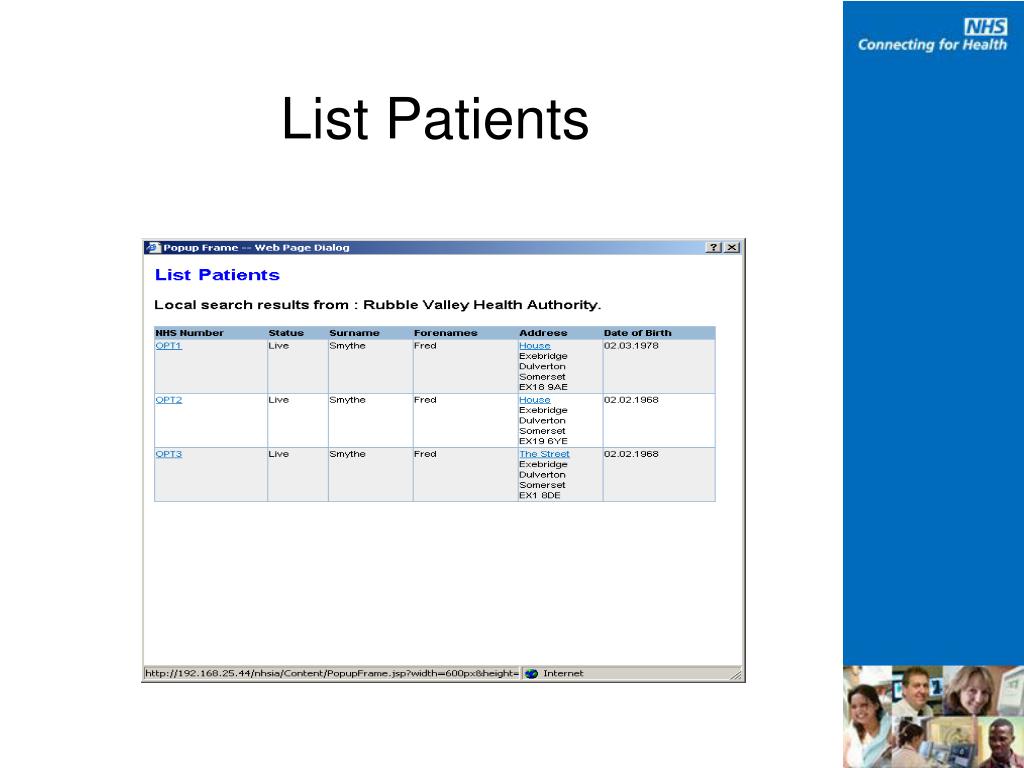The image features a detailed screenshot of a computer interface with a white background and several distinct sections. Dominating the upper portion of the image, "List Patients" is prominently written in black text. Below this title, the central area displays a screenshot of a web page interface, featuring a popup window labeled "popup frame, web page dialogue." This section shows a grid layout with columns categorized by NHS number, status, surname, forenames, address, and date of birth in varying shades of gray and white. The grid includes specific patient details under "Local Search Results from Coleman-Rubble Valley Health Authority."

On the right side of the image, a vertical blue sidebar is present, featuring the NHS (National Health Service) logo and the phrase "Connecting for Health." At the bottom of the image, there is a small collage of thumbnail photos showing a diverse group of five individuals, including at least one Black person and a few Caucasian people. One of these thumbnails shows a woman examining computer monitors. Overall, the entire composition is set against a white background, creating a clean and clinical visual presentation.